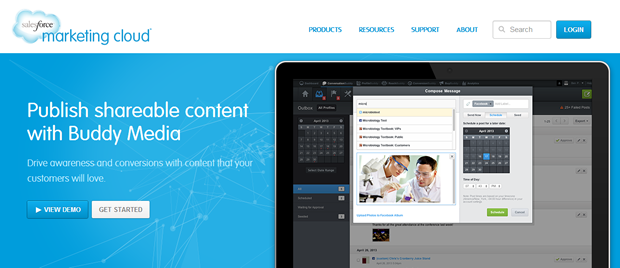On the left-hand side of the image, there is a white background reminiscent of clouds in waves, with "Salesforce" written in black text outlined in blue. Adjacent to this, "Marketing Cloud" is displayed in bold blue text, followed by options labeled "Product," "Resources," "Support," and "About" in blue font. A white search box outlined in gray, complete with a gray magnifying glass icon and the placeholder text "Search," is also present. To the right of the search box, a blue rectangle features the word "Login" in white text.

The background transitions into a blue gradient with faded white lines and a message in white text that reads "Publish shareable content with Buddy Media. Drive awareness and conversions with content that your customers will love."

Below this message, there are two rectangular buttons: the first is blue with a white play icon and the text "View Demo," while the second is gray with darker gray text that says "Get Started."

On the right side of the image, there appears to be the top part of a device, possibly a tablet or a desk, framed in black and silver. The text on this device is blurry but seems to read "Compose Message." Additionally, there are two people wearing lab coats and goggles standing near a white microscope with a black base. The scene is enclosed in a clear, blue-tinted frame.